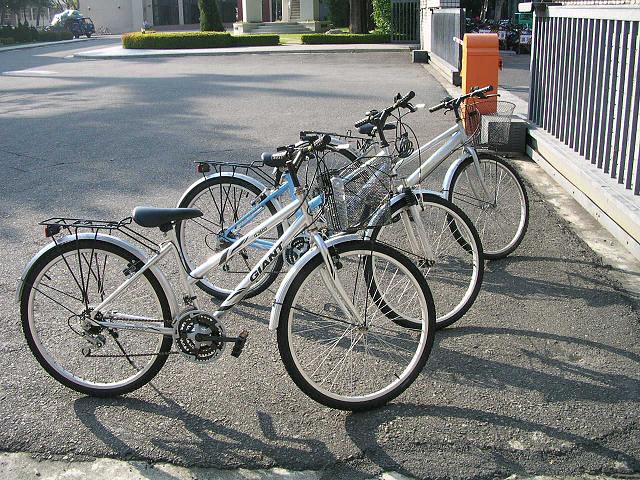In a bright daytime outdoor photograph, three brand-new bicycles are parked in a row on a macadam parking lot, their front tires pointing to the right. Each bike features spoked wheels, black tires, predominantly white frames with one having hints of blue, black handlebars, black seats, and chrome fenders at both the front and back. All the bicycles are equipped with flat, metal racks over the rear tires. The sunlight coming from the upper left casts shadows on the right side of the bicycles, emphasizing their sleek, almost pristine appearance. The down tube of each bike frame is marked with the brand "GIANT" in bold black letters.

The scene also captures the fenced perimeter to the right of the bicycles, with an adjacent red and white gate arm, and an orange gate post visible near the entrance. In the distant background, partially obscured by shadows and sunlight, a building is nestled behind a neatly trimmed hedge. Further right, a sidewalk and some short greenery lead up to the building, while on the far left, a parked vehicle peeks out from behind some bushes, adding to the context of this well-composed display.